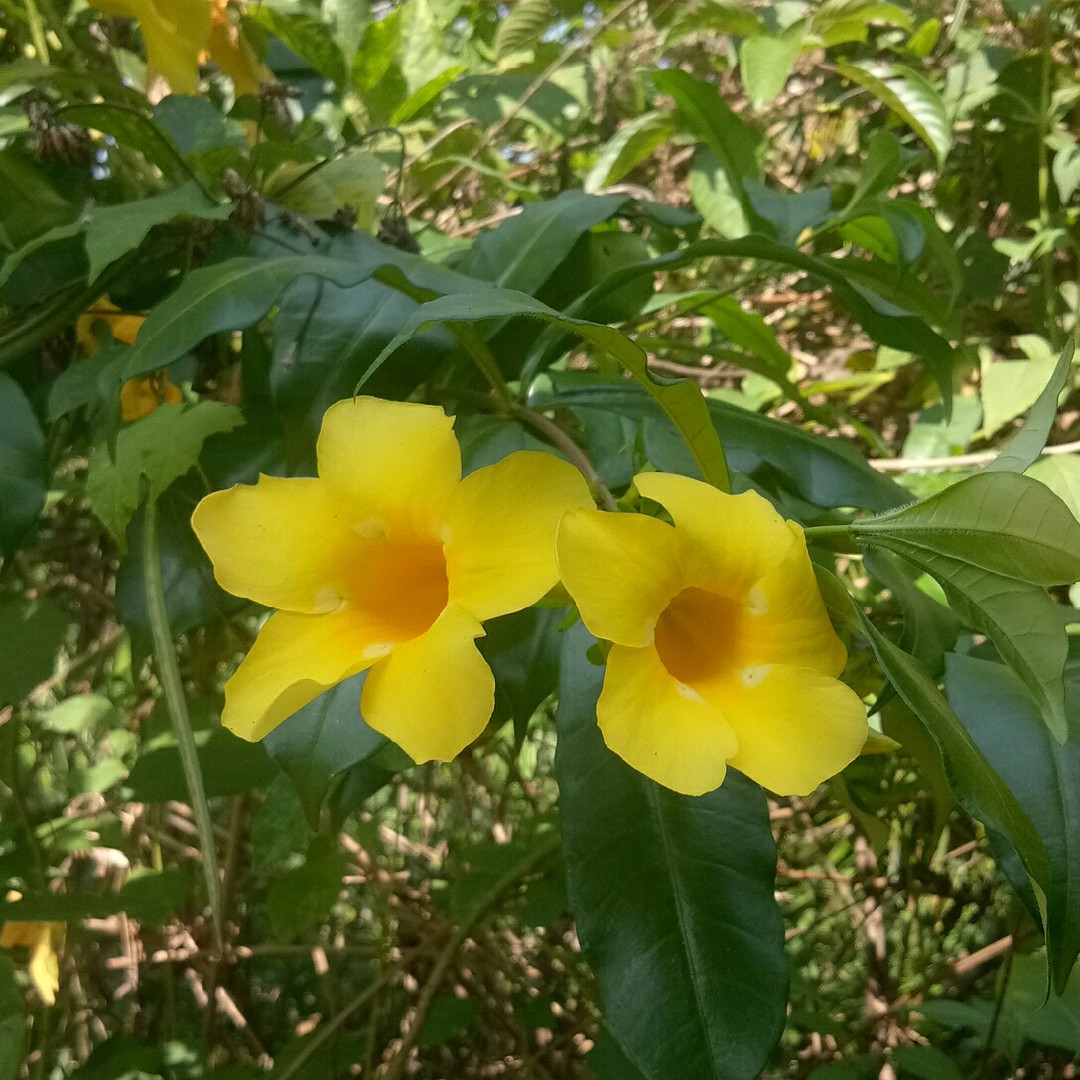The color photograph depicts a dense outdoor shrubbery scene under bright daylight. Central to the image are two vibrant yellow, tubular flowers resembling Carolina jasmine, though this plant appears more shrubby than vine-like, with glossy, deep green, long leaves. The flowers flaunt five petals each, radiating a sunny, lemon-yellow hue, and possess deep yellow throats, ideal for attracting hummingbirds. In the background, a lush tangle of greenery and stems can be observed, alongside scattered details such as dry grass and, notably, a pine cone in the top left. The foreground flowers are positioned in a shaded contrast to the sunlit backdrop, where light filters through, illuminating the tops of the surrounding leaves. This photorealistic capture features no text, emphasizing the natural beauty and complexity of the scene.